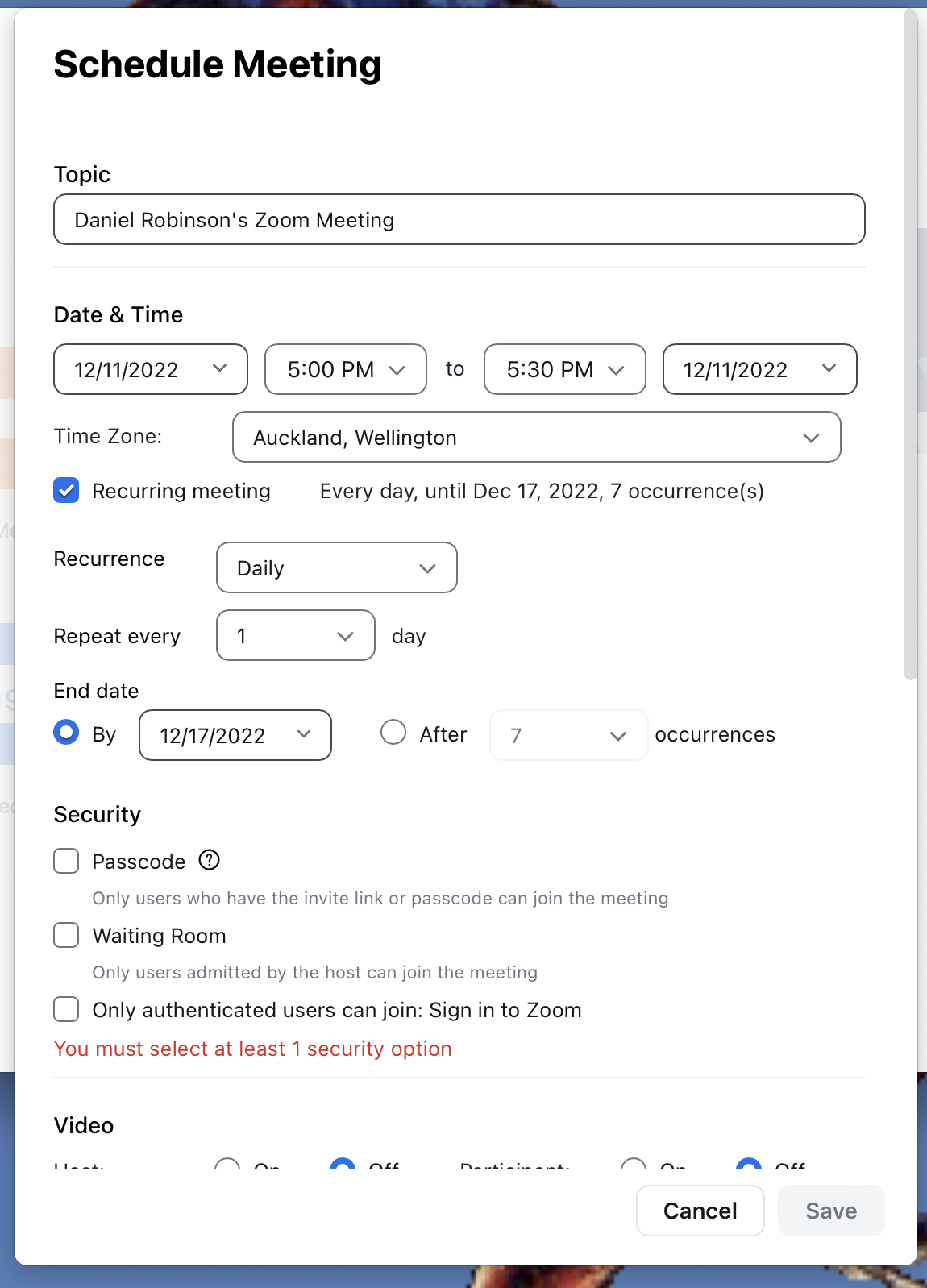The image is a screenshot of a "Schedule Meeting" page from a Zoom interface, detailing the setup for Daniel Robinson's Zoom meeting. 

At the top of the page, it prominently displays the title "Schedule Meeting." The first visible text field is labeled "Topic" and contains the entry "Daniel Robinson's Zoom meeting." Below this, there are dropdown fields for selecting the meeting's date and time. The current selections are set to December 11, 2022, from 5:00 PM to 5:30 PM. Another dropdown field shows the time zone, which is set to "Auckland-Wellington."

A check mark is placed next to the "Recurring Meeting" option, which specifies that the meeting will occur daily until December 17, 2022, totaling seven occurrences. The recurrence pattern is further defined by a dropdown labeled "Occurrence," set to "Daily," and another dropdown labeled "Repeat," set to "Every 1 day." Additionally, a radio button under the "End Date" section notes that the recurring meetings will end by December 17, 2022.

Below these settings, there are three security options—each with corresponding checkboxes—but none are currently selected. The options available are "Passcode," "Waiting Room," and "Only Authenticated Users Can Join: Sign in to Zoom."

This organized layout allows comprehensive customization for scheduling and securing Zoom meetings.